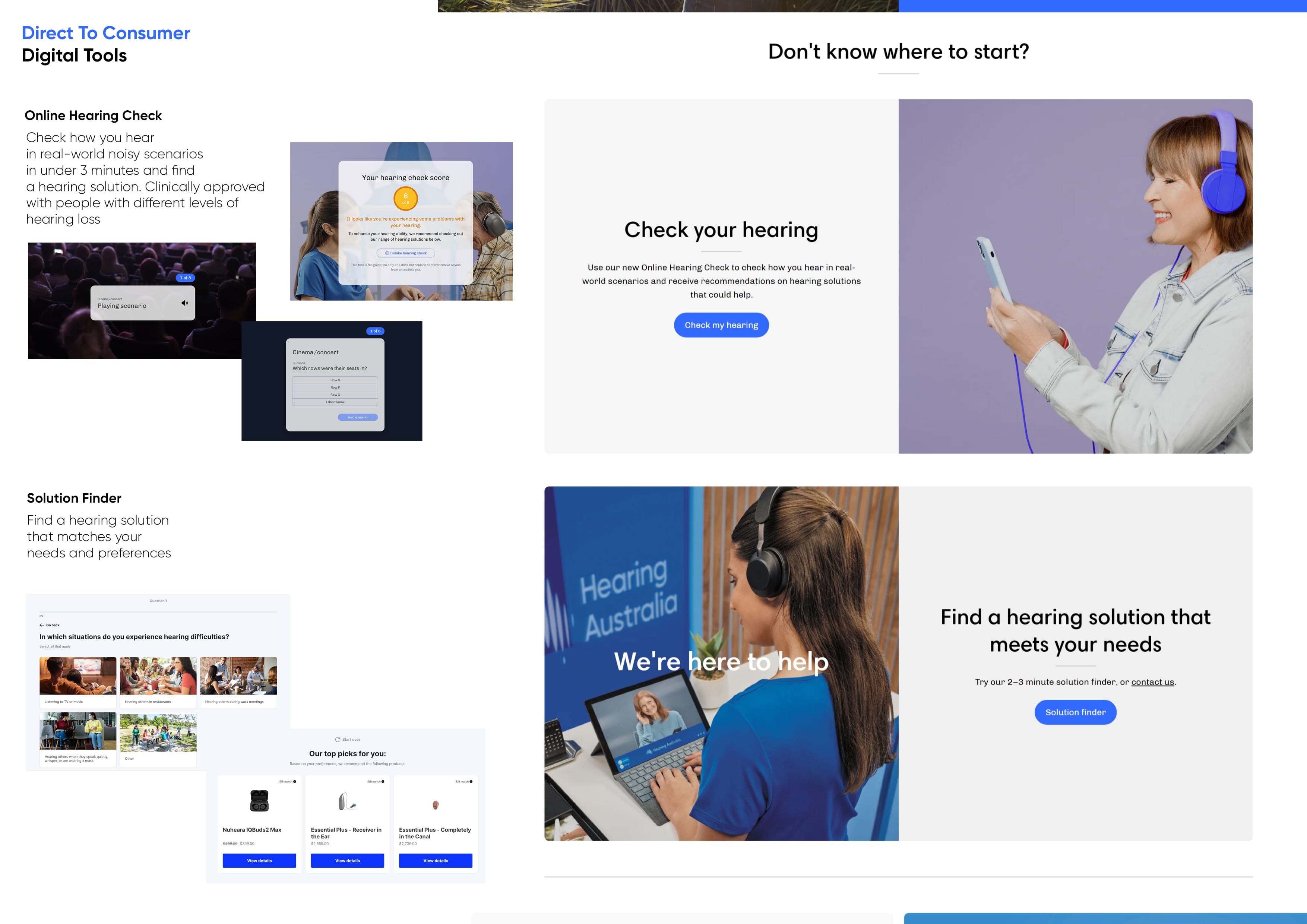The image showcases a web page with a clean, white background, featuring a visually appealing collage of various images and texts arranged in square and rectangular frames. In the upper right corner, the text "Don't know where to start?" is prominently displayed in black. Below this text, a smiling woman wearing a light-colored denim shirt and blue headphones is visible. She holds a white device with a dark blue cord in her hand. To the left of this image, the phrase "Check your hearing" is written, accompanied by smaller text and a distinctive blue oval button. Further down, another image shows a woman facing away, dressed in a blue t-shirt and also wearing blue headphones. In white text printed across the front of this second image, it reads, "We are here to help."